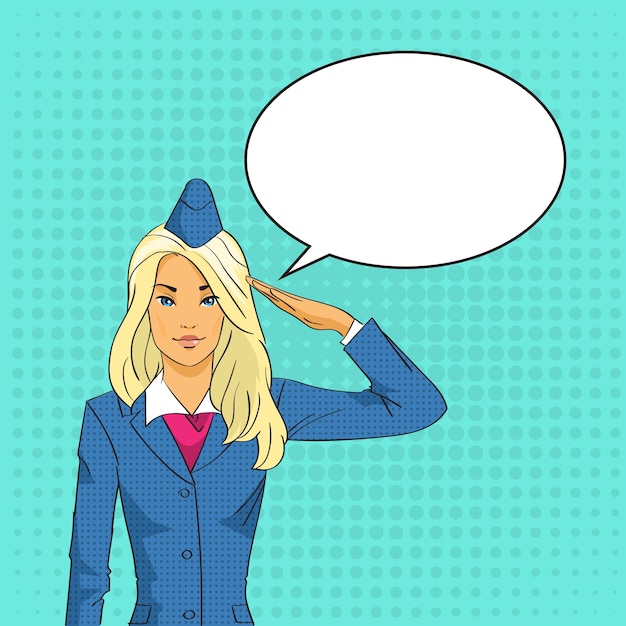The image is a cartoon drawing of a Caucasian woman, likely a flight attendant, dressed in a uniform. She has long blonde hair cascading to just below her armpits and striking blue-green eyes. Her attire consists of a navy-pilot-blue outfit with a wide white collar and a pink ascot underneath. The uniform features three buttons down the front and pockets with flaps just at her waistline. She is wearing a matching blue pointed cap adorned with small blue dots and is seen smiling while looking directly at the viewer. In the image, she is performing a salute with her left hand while her right arm rests by her side. The background is an aqua green with polka dots increasing in size towards the center, creating a gradient effect. Positioned off to the right, above her hand, is a white speech bubble outlined with a black line, which is currently blank. The woman is standing to the left of the center of the image.